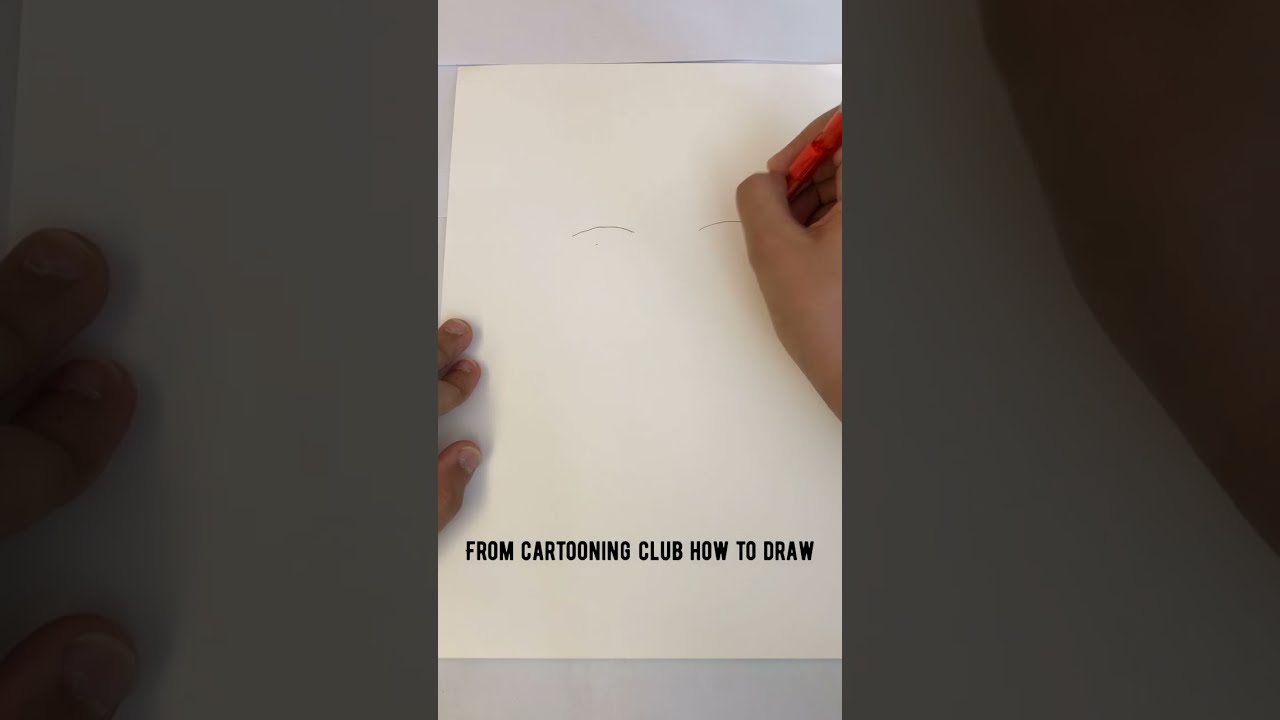In this detailed image, a person with short-cut fingernails and dark complexion is beginning to draw on a white piece of paper that lies flat on a table. The central focus is the paper, prominently displaying the black capitalized text "From Cartooning Club, How to Draw" at its bottom, likely superimposed. The artist is using an orange-red pencil with some indistinguishable markings on it, held in their right hand, as they begin sketching what appear to be eyebrows—thin, curved lines resembling the tops of ovals. The left hand is partially visible, with only a few fingers seen near the left edge of the paper. The close-up view in the image reveals the base of the person's palm on the top right and three fingers on the bottom left. The white background, combined with the scattered colors of gray, brown, and black, along with the textured orange-red pencil, suggests that the setting is part of an instructional video, possibly shared on social media platforms like TikTok or Instagram, aimed at teaching cartoon drawing techniques.